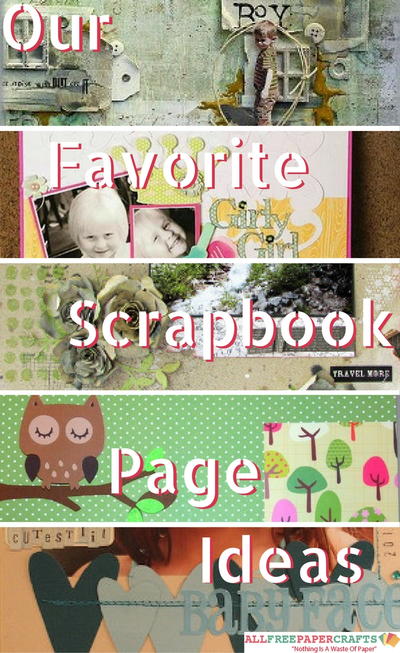The photograph is of a book cover adorned with a collage of various rectangular pictures and illustrations, meticulously arranged into five distinct sections from top to bottom. At the top, the book cover features the text "Our Favourite Scrapbook Page Ideas" in white, encapsulated by a red border. The uppermost section showcases a picture of a boy with a green background and the typewritten letters "R-O-Y" in black above his head. Just below, the second section contains smiling kids against a brown background, and the word "Favourite" is prominently displayed in white with a pinkish outline. The central area features an abstract floral design with an evocative image of a waterfall, labeled "Scrapbook." The fourth segment presents a green polka dot background dominated by a brown owl perched on a tree branch, alongside the word "Page." Finally, the bottom section portrays an abstract depiction of a woman's neck set against a beige backdrop, coupled with black and gray heart cut-outs and the word "Ideas." This intricate and layered design theme is visually rooted in the conceptual style of scrapbooks.